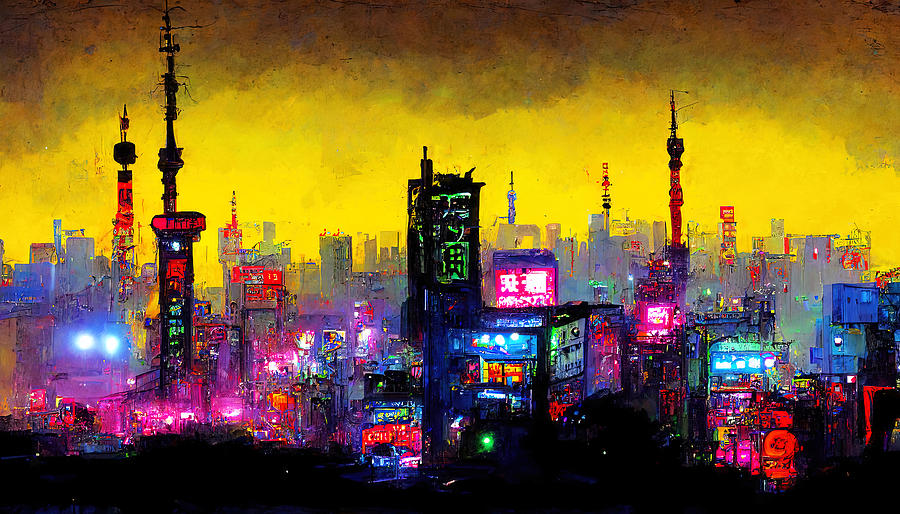This image is a vivid, stylized painting of a sprawling, futuristic cityscape illuminated by an array of neon lights. The scene is viewed from a slightly elevated angle, offering a sweeping look across the densely packed buildings. The sky forms a striking backdrop, transitioning from a dark brownish-black at the top to a bright, golden yellow near the horizon. Dominating the foreground is a labyrinth of towering structures, adorned with bold neon hues of pink, blue, green, and red. The buildings, some of which fade into the background with hints of gray, red, and blue, feature numerous signs that appear to be written in an Asian script, adding a cultural touch to the futuristic theme. Amongst the urban jungle, a particularly tall and slim structure with a radio tower stands out on the left, painted in red and black, while central to the image is a blue-lit building topped with a pink roof and more Asian script. Another tall building with green adornments is situated behind it, accompanied by additional towers strewn with pink lights on the right. The very bottom of the image is shrouded in ominous black shades, suggesting shadowed structures or open spaces, enhancing the city's enigmatic allure.